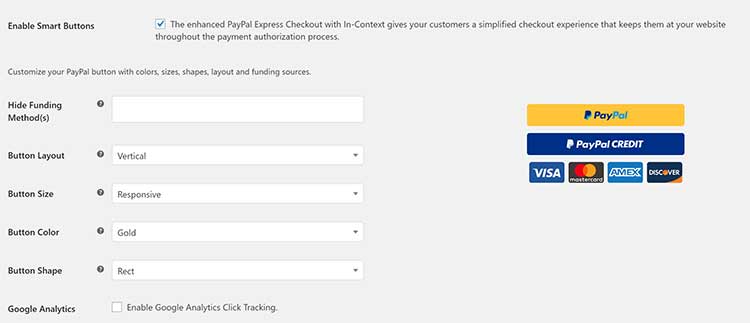A detailed desktop screenshot showcases a user interface with settings for customizing PayPal buttons. The background is light grey with black text for easy readability. At the top, the text reads, "Enable smart buttons," accompanied by a checked checkbox. Below, a description states, "The enhanced PayPal Express checkout within context gives your customers a simplified checkout experience that keeps them at your website throughout the payment authorization process."

Further down, the text explains, "Customize your PayPal button with colors, sizes, shapes, layout, and funding sources." Here, several customization options are presented:

1. **Hide funding methods** – accompanied by a blank entry bar.
2. **Button layout** – showcased with a drop-down menu currently set to "Vertical."
3. **Button size** – showcased with a drop-down menu currently set to "Responsive."
4. **Button color** – showcased with a drop-down menu currently set to "Gold."
5. **Button shape** – showcased with a drop-down menu currently set to "RECT."

Each of these customization options is accompanied on the left side by a small black icon featuring a white question mark for additional help.

Underneath all these customization options, there is a setting for Google Analytics, including an unchecked checkbox labeled, "Enable Google Analytics click tracking."

On the right side, isolated from the rest of the text and customization options, there is a set of buttons:
- A long rectangular yellow button labeled "PayPal"
- A blue button labeled "PayPal Credit"
- Four images depicting logos of different credit card companies.

This comprehensive layout allows for extensive customization and integration options for PayPal and related services.